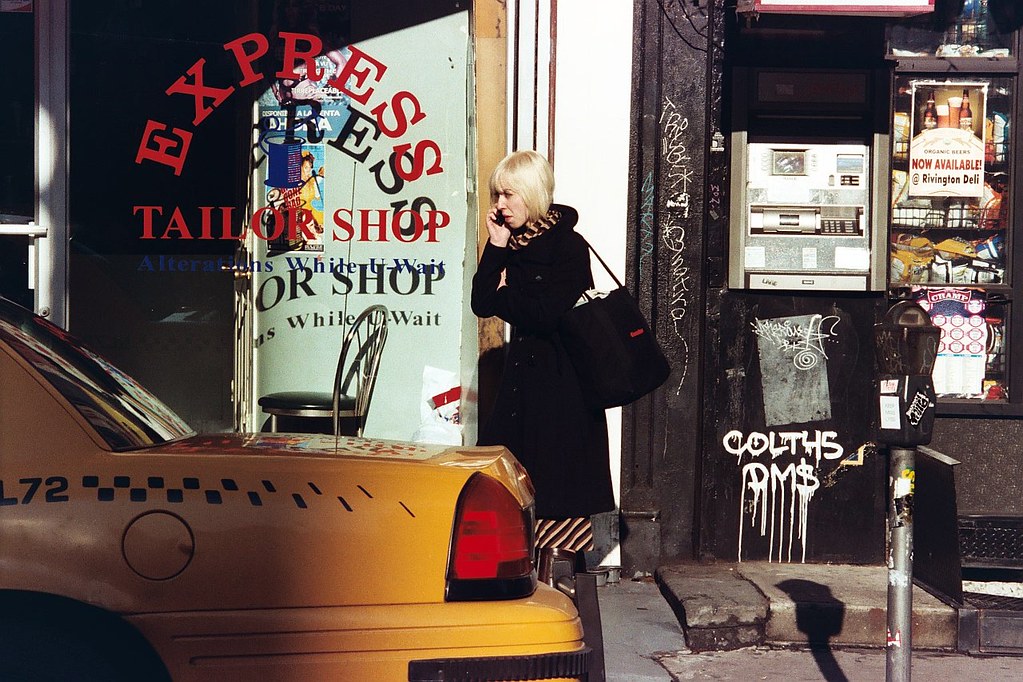In an urban downtown setting, a young blonde-haired woman stands at the center of the image, slightly turned to her left, around the nine o'clock position. She is dressed in a long black coat over a striped black, tan, and brown dress, and carries a black bag on her left arm, while holding a cell phone in her right hand. She leans slightly against the front of the Express Tailor Shop, which is marked by a dark appearance, large window with a single black metal chair, and signage in red and blue script.

The scene behind her includes an ATM built into the shop wall, heavily marked with white graffiti and tags like "Kohl's" and "DMS." Directly right of the ATM in a grimy display window of what appears to be a convenience store, there are beer bottles. A worn-out parking meter, covered in stickers and graffiti, stands closer to the foreground. The sidewalk beneath her feet is visibly cracked and shows signs of neglect. Additionally, the rear end of a bright yellow taxi cab is visible off to the left, hinting at the bustling urban environment surrounding her.